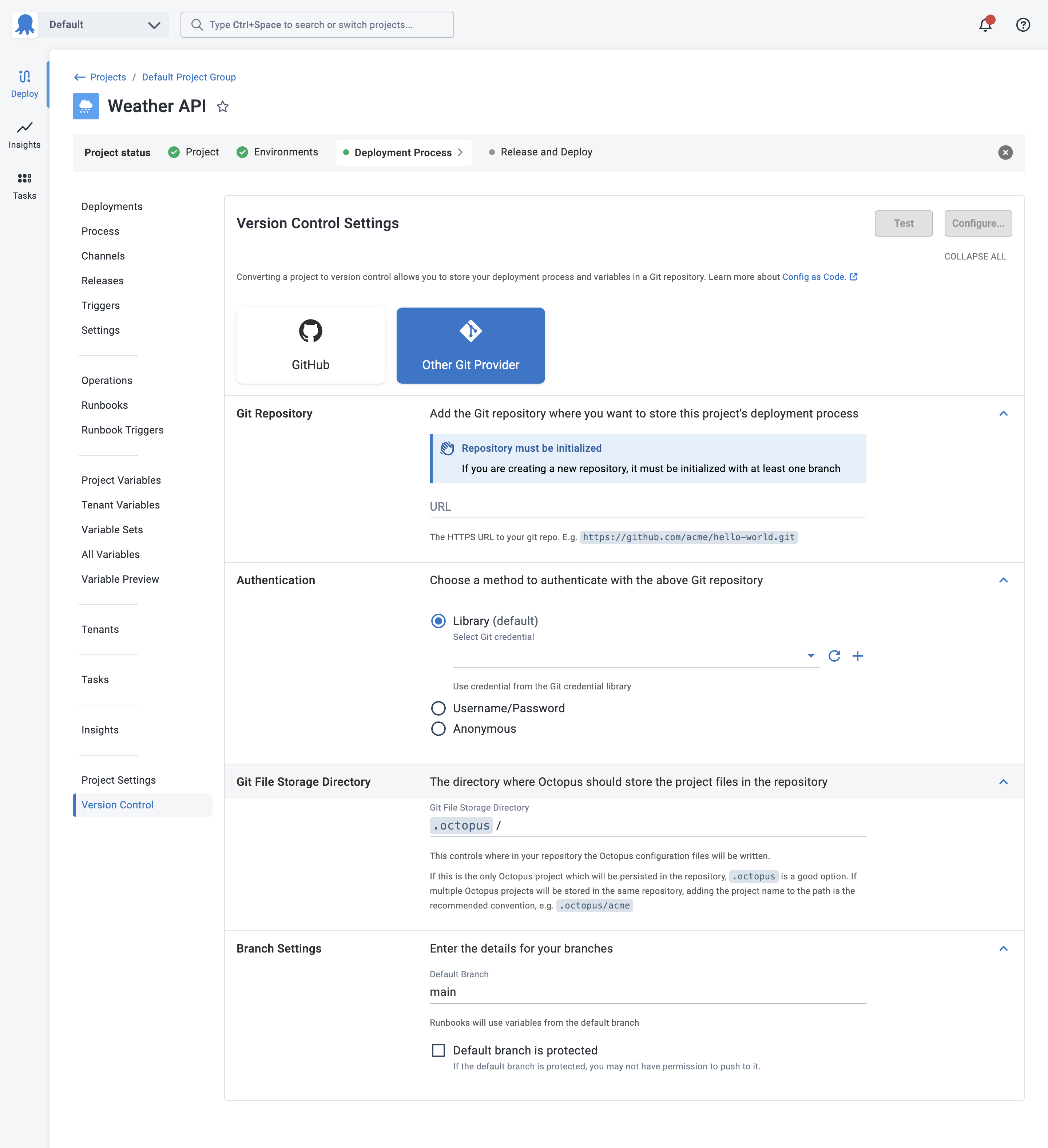The image appears to be a screenshot of a computer screen displaying a management dashboard interface. At the very top of the image, there is a navigation bar featuring several sections: "Default" in black on the upper left, followed by "Dashboard" in blue, and then "Projects," "Infrastructure," "Tenants," "Insights," "Library," "Tasks," and "More." To the right of these sections, there is a small search area, a white bell icon, and the label "Octonaut."

Below the "Default" section on the left side, the interface lists several categories under the "Projects" heading. This includes "Project Group," with a list underneath featuring options like "New Project," "Create," and "Release." The "Deployments" category is also listed, and it has sub-sections such as "Overview," "Process," "Channels," "Releases," "Triggers," and "Settings." Additionally, the "Operations" section is visible with sub-sections for "Overview," "Runbooks," and "Triggers." Other categories listed on the left include "Variables," "Tasks," "Insights," and a "Settings" section which contains "General" and "Version Control."

In the center of the image, it is evident that the "Version Control" settings have been selected. At the top of this section, there is an entry for "Git Repository," followed by a section for "Authentication," a "Git File Storage Directory," and a "Branch Settings" section. The overall layout indicates a detailed project management system with various navigational and functional tools centralized on this interface.